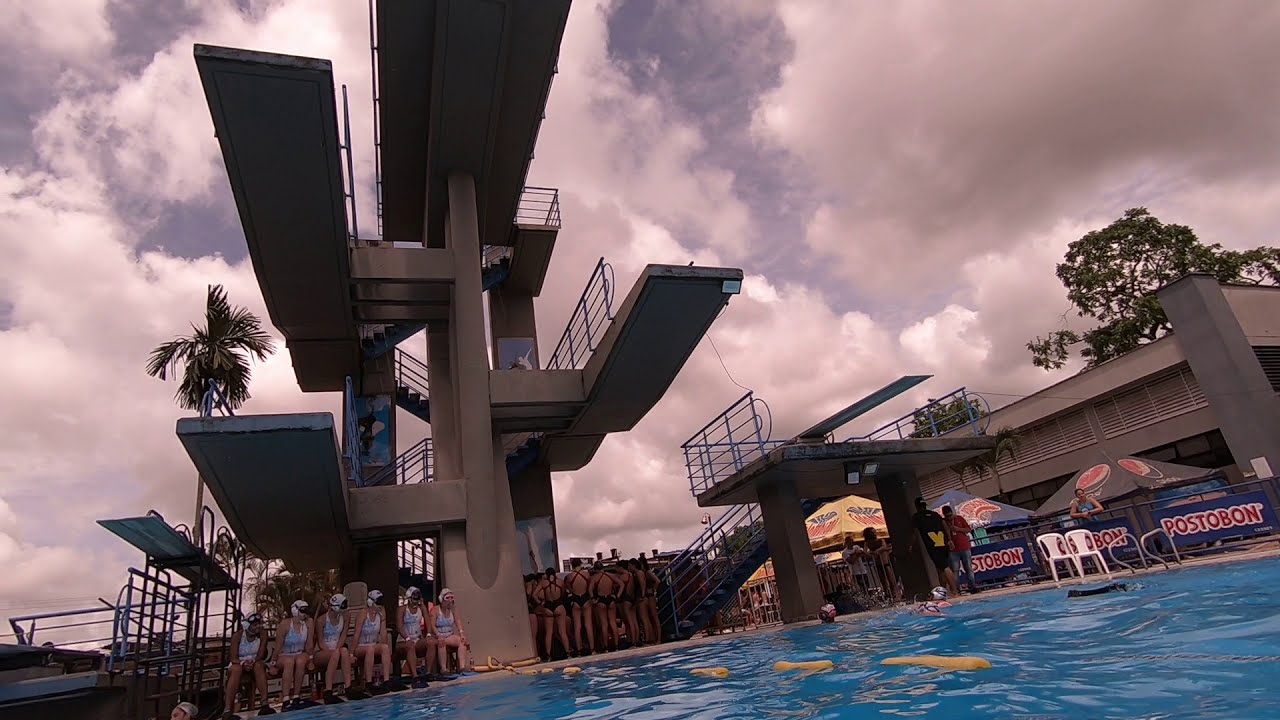This detailed photograph captures the bustling scene of a large swimming pool area, likely set at a competitive event or swim park. The vantage point from the middle of the pool showcases its vibrant blue water and the clear blue sky dotted with white clouds. The pool is divided by a yellow floating divider, and the surrounding areas feature the word "PASTOBON" repeatedly displayed in red and white letters against a blue background.

Outside the pool, there are numerous elevated platforms and multiple diving boards from which participants can jump. The teams are distinctly dressed, with one group in black swimsuits and another in white, indicating a competition. Various young swimmers, both male and female, are gathered in different spots, some wearing swim caps. One group is seated on chairs, while another is standing and discussing strategies.

To the left, a tall palm tree adds a touch of tropical flair, and on the right, a deciduous tree stands behind a building, creating a contrast in greenery. White plastic chairs are scattered around, and a few people are seen walking back and forth. A building with awnings or umbrellas bearing designs and advertisements is visible on the right, enhancing the lively, organized environment.